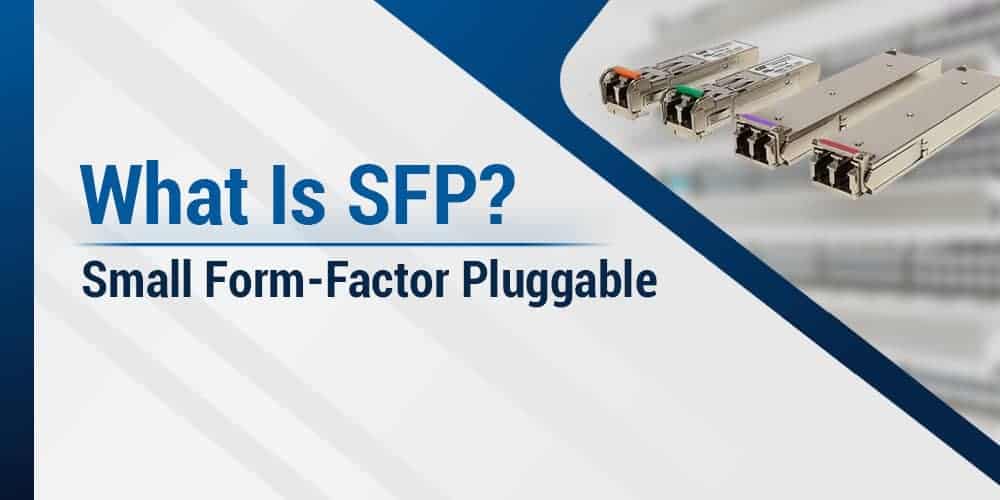The image appears to be a detailed diagram from a brochure or presentation about an electronic device called Small Form-Factor Pluggable (SFP). It features a blue and white color scheme with a prominent heading in dark blue letters that reads, "What is SFP?" followed by a blue line separator. Underneath the heading, in dark blue letters, it states, "Small Form-Factor Pluggable," with the acronym and its expansion clearly defined. 

On the right side of the image, there are four rectangular, metallic devices displayed, each fitted with a tiny cylindrical piece on top. These devices are differentiated by distinct color-coded bars: one orange, one green, one purple, and one red. The background includes a light gray triangular overlay and a white half-square area with some gray mix, adding to the visual structure. The diagram effectively combines textual information with visual aids to explain the concept of SFP modules.